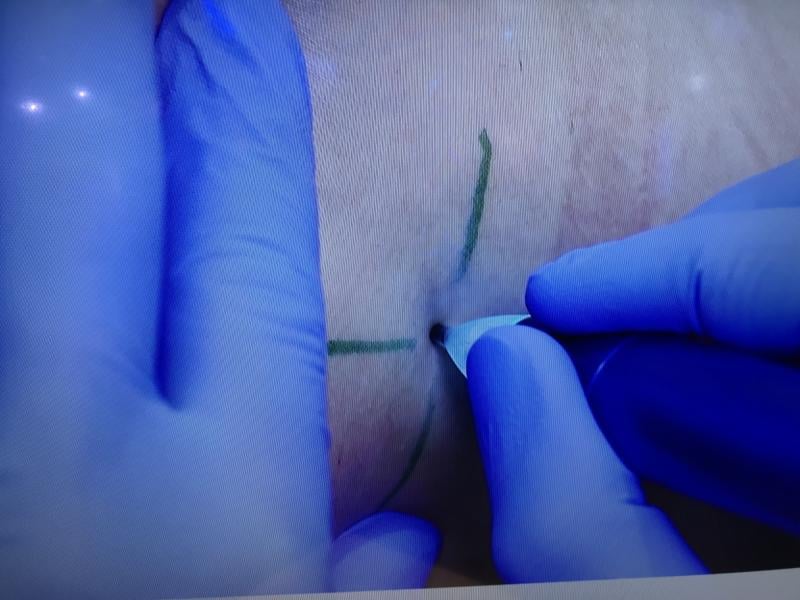The photograph captures a detailed, close-up view of a medical procedure being performed indoors. The focal point is a section of a person's skin, likely the lower abdomen or a similarly flat and fleshy area, marked with a green T or X shape. This marking seems to guide the precise point of insertion for the device being used.

Two hands, adorned in blue surgical gloves, dominate the image. The left hand, visible in the left side of the image, is seen holding the skin firmly, with clear view of the thumb, index, and middle fingers. The right hand, emerging from the lower right corner, manipulates what appears to be a pen-like instrument with a blue handle and a sharp white tip. This tool, potentially equipped with a lighted tip, is being carefully pushed into the skin at the juncture of the green markings.

The skin, showing visible veins and lines, suggests a Caucasian individual. Reflections from two overhead lights add more illumination to the scene, highlighting the meticulous nature of the procedure.